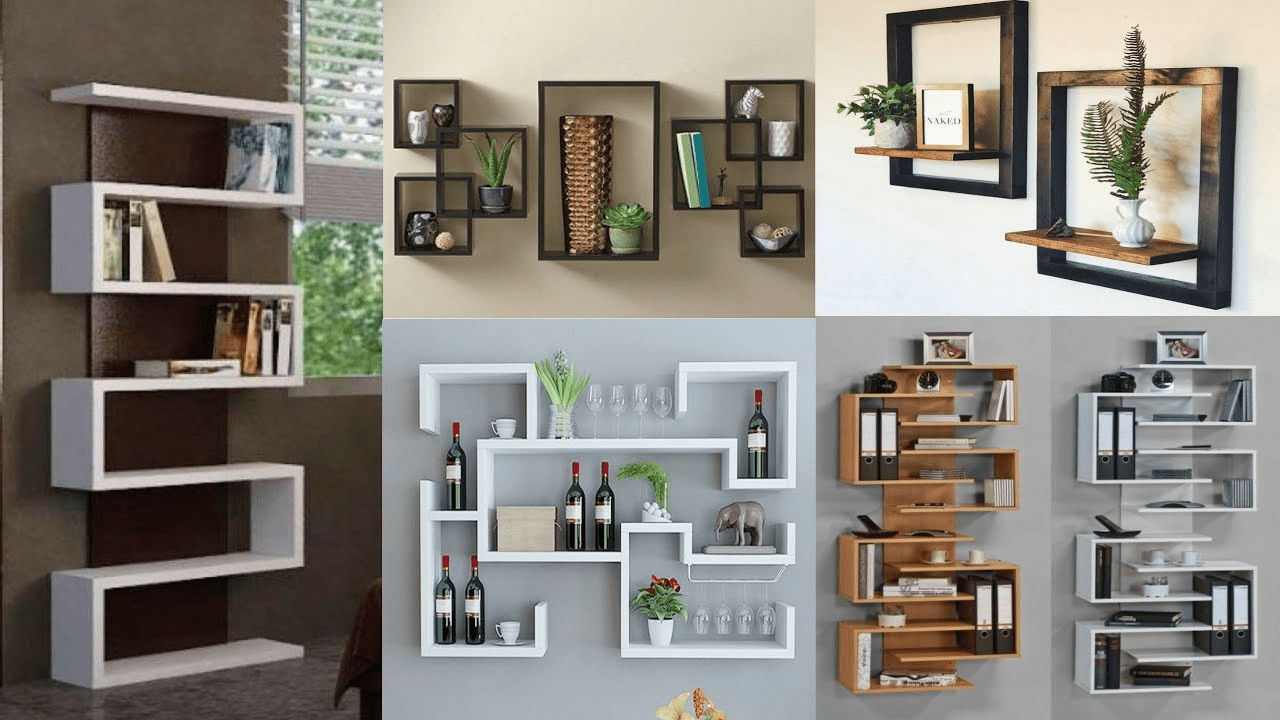This image is a detailed collage of five distinct photographs showcasing various contemporary wall shelving units on different colored walls. 

- The leftmost photograph occupies its own vertical space and features a white, zigzag-patterned shelf resembling a sequence of the number two joined together, mounted on a dark brown wall. This shelf holds a few books and is partially framed by white window blinds with a tree visible outside.

- The upper left quadrant of the collage displays black, open rectangular and square shelves on a beige wall, adorned with potted plants and other décor items.

- The upper right quadrant showcases two black frame-like units with wooden shelves extending from them, each holding small potted plants.

- The bottom left section includes a uniquely shaped white shelving unit with multiple compartments, resembling a somewhat rectangular but complex geometric form. This shelf accommodates wine bottles, wine glasses, an elephant figurine, and some plants.

- Finally, the bottom right quadrant mirrors the first section's zigzag pattern but in two separate shelves—one white and one tan. They hold various items including larger books, teacups, clocks, and picture frames, illustrating the versatility of the shelving designs.

Together, the collage provides a comprehensive view comparing different modern and geometric wall shelving solutions suitable for various interior décors.